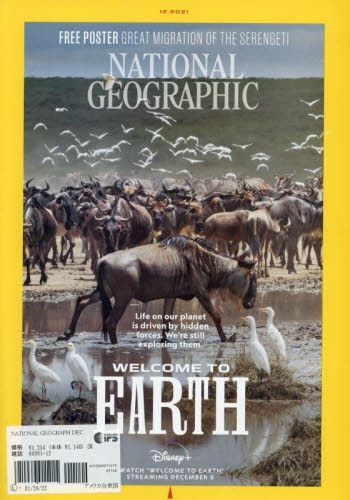This captivating photograph features the cover of a National Geographic magazine from 2021. The iconic yellow border encircles the cover, affirming its authenticity, along with a discernible price tag in the lower left-hand corner, although the exact price remains illegible. Dominating the cover is a stunning image of water buffalo surrounded by white birds in flight and scattered muddy puddles, capturing the raw beauty of the Serengeti's great migration.

Prominently positioned beneath the photograph, the text reads: "Life on our planet is driven by hidden forces. We're still exploring them." An eye-catching, large font at the bottom declares, "Welcome to Earth," accompanied by an ad for the Disney series "Welcome to Earth," streaming from December 8th. Interestingly, the price sticker appears to be part of the cover design, cleverly skewed at an angle behind the text of the "E" in "Earth," adding an intriguing, almost playful element to the composition.